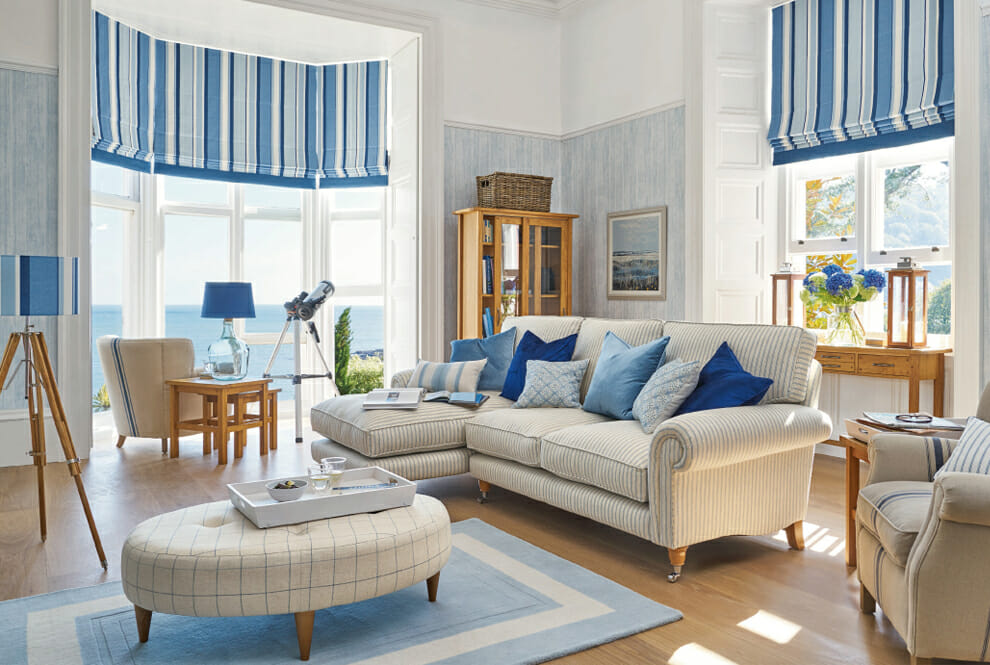This photograph showcases a serene living room interior bathed in daylight, with a soft color palette predominantly featuring shades of blue, white, and light-colored wood. The left side of the room is defined by a large bay window offering a stunning view of clear blue water, possibly the ocean. Adjacent to it, on the right, is a smaller square window providing a glimpse of trees and a mountain range. The center of the room boasts a pale blue area rug beneath a round white footstool that serves as an ottoman, topped with a white tray holding a bowl of food and a couple of glasses. To the right of this setup is a white couch adorned with light gray stripes and an array of variegated blue throw pillows. Near the couch, there are two overstuffed armchairs, each accompanied by an end table holding blue-shaded lamps. 

In one corner, a large wooden curio cabinet with glass doors showcases various objects, with a wicker basket placed on top. The right side of the image captures a vase of blue and white hydrangeas positioned near the small square window. Adding to the room's tranquil atmosphere is a telescope positioned by the bay window, though the sunny view outside makes it unnecessary at the moment. The walls lower parts are painted light blue, complementing the aqua and white striped rug that covers part of the wooden floor. Additionally, a painting adorns one of the walls, adding to the room's decorative elements.